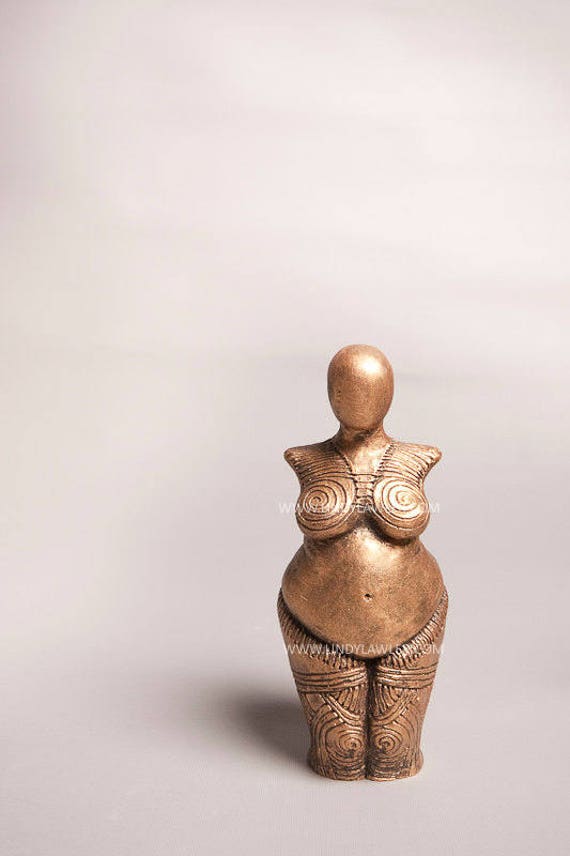This photo showcases a bronze or copper-colored fertility goddess statue set against a tall, light to dark grey background. The statue, evocative of a classic Venus figure, is positioned at the bottom right of the image. With an oval-shaped and featureless head, the statue lacks facial details, arms, and legs below the knees. The figure displays pronounced breasts adorned with spiral designs, and decorative patterns extend down the legs, suggesting pants or similar attire. The curvaceous body captures the essence of an ancient artifact, embodying a female form with exaggerated features conveying themes of fertility and womanhood.